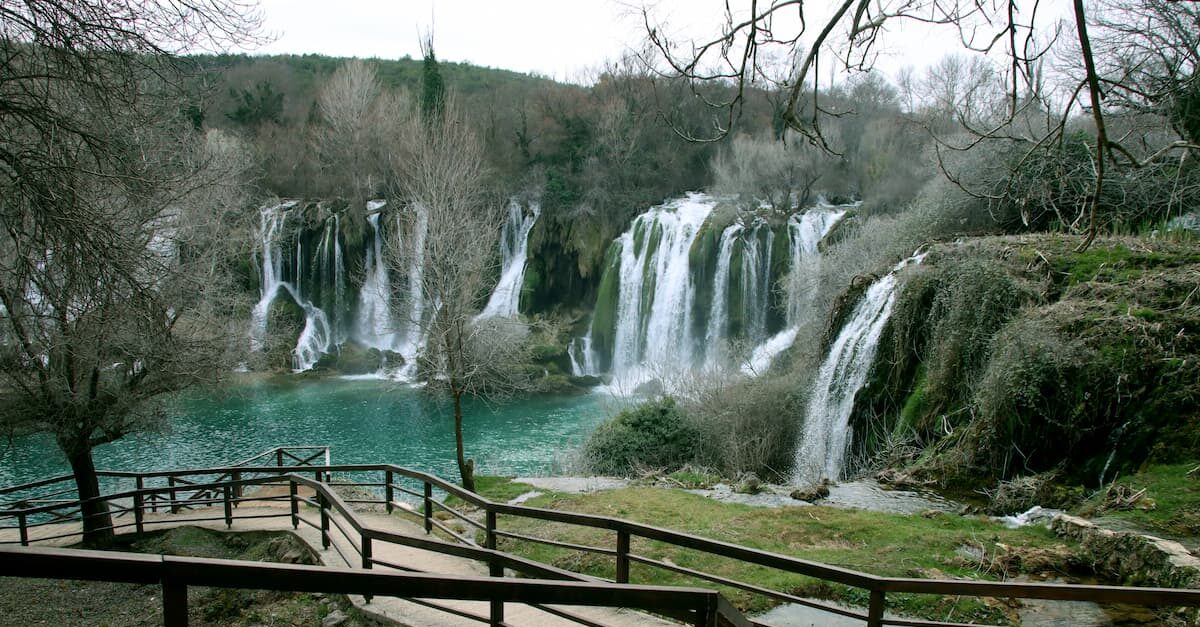In this color outdoor photograph of a picturesque park, a series of small waterfalls and streams cascade down green, grassy hills into a tranquil, green-hued body of water. The scene is surrounded by a lush mix of trees, many of which are barren and without leaves, suggesting the season could be fall. 

In the foreground, a brownish metal railing lines a cement ramp and wooden walkways that wind down from the photograph's viewpoint to the lower level where the waterfalls combine into the serene pond or small lake below. The multiple waterfalls create a serene and inviting atmosphere, perfect for a remote vacation spot. The lush greenery and rustic pathways meander through the landscape, highlighting the natural beauty and peacefulness of the setting.